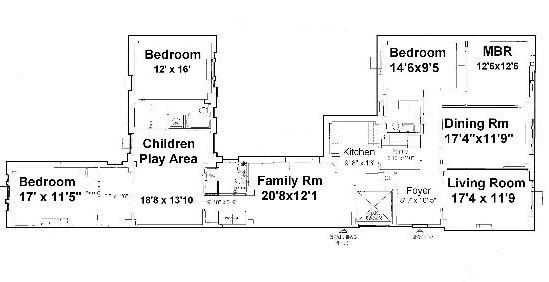The image illustrates a detailed black-and-white floor plan. On the far left, there is a spacious bedroom measuring 17 by 11 feet. Adjacent to this bedroom, directly to the right, is a children's play area encompassing 18 by 13 feet. Above the play area, there is another bedroom with dimensions of 12 by 16 feet. Next to the children's area lies a generous family room, sized at 20 by 12 feet. To the right of the family room, there's a partially blurred kitchen area that appears smaller in comparison to other rooms; its exact measurements are unclear.

Continuing right from the kitchen, you encounter a foyer. Adjacent to the foyer, on the right, is the living room, which measures 17 by 11 feet. Above the living room is a dining room of the same dimensions, 17 by 11 feet. Above the dining room, you will find the master bedroom, featuring a size of 12 by 12 feet. Additionally, there is a second bedroom above the dining room, which measures 14 by 9 feet. The floor plan does not distinctly show any bathrooms, possibly obscured in the blurred sections.